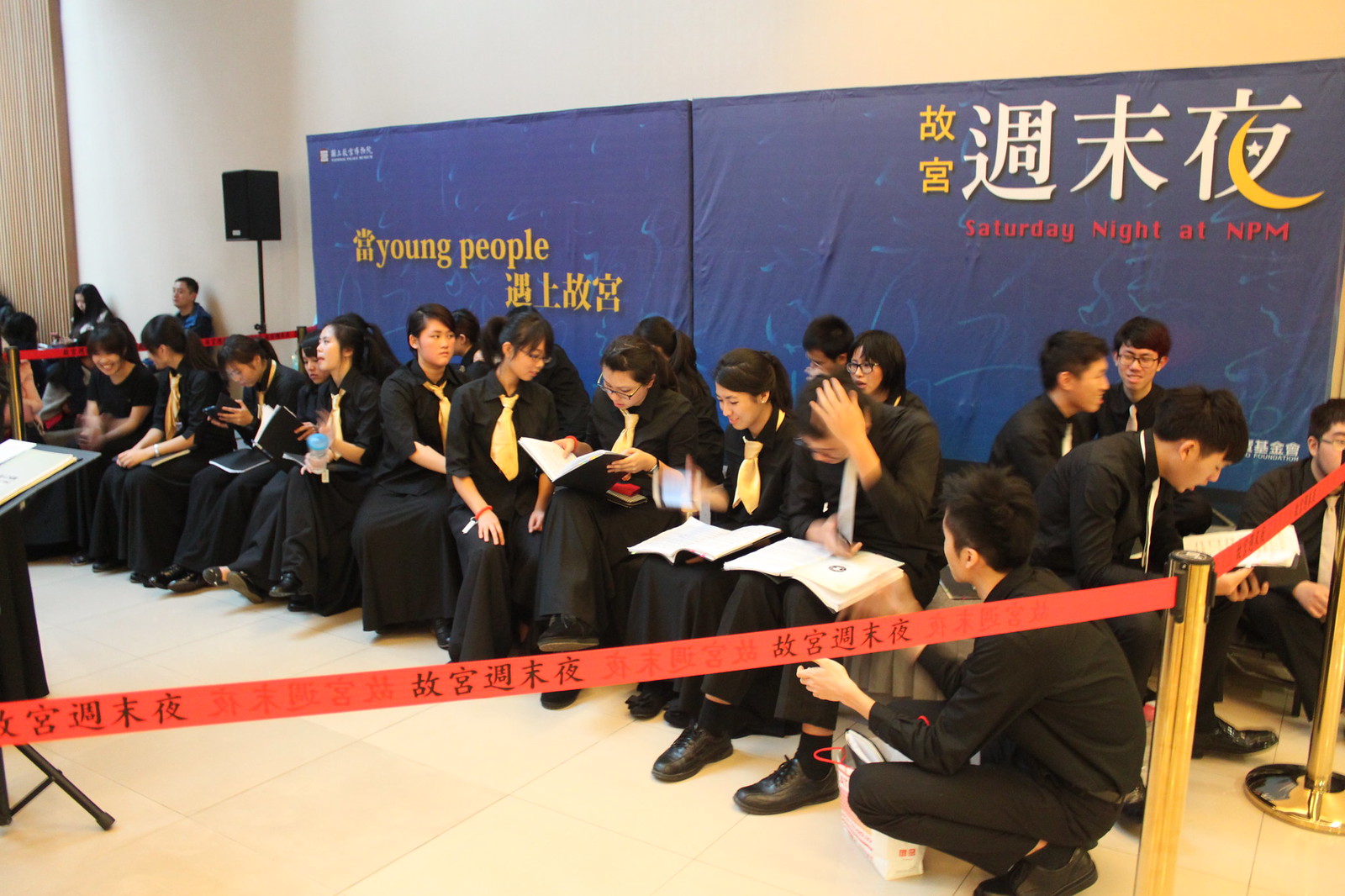The image captures a graduation ceremony for Japanese college students, where the attendees are dressed in black attire, including black shirts, trousers for men, and black skirts for women, all complemented by yellow ties. The students are seated or kneeling on a cream-colored tile floor, with a red ribbon held up by gold posts cordoning off the area, reminiscent of a police barrier. Surrounding them are notable features: on the far left, a music stand or lectern with an open book, and in the background, a large black speaker and some people sitting in a corner. Dominating the backdrop are two giant blue scrolls, one inscribed with "Saturday night at N.P.M." in white and yellow, and "young people" in yellow, mixed with Japanese writing. The scene conveys a solemn yet celebratory atmosphere, with the students appearing contemplative, possibly preparing for a speech or a significant examination.